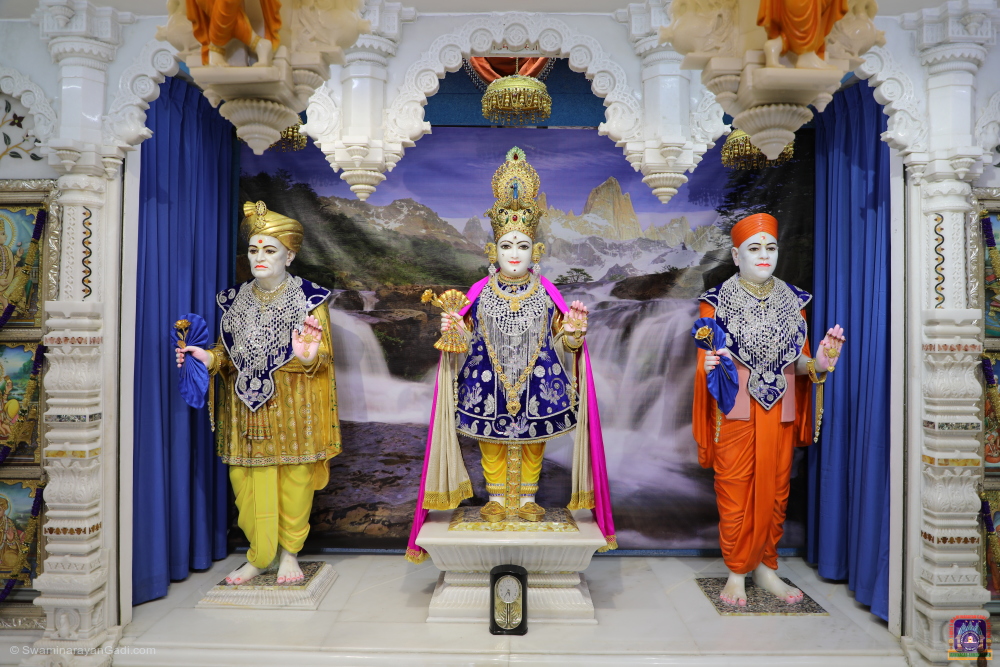The image displays a vibrant and ornate setting with three porcelain statues, each distinctively dressed, standing on a pedestal. The backdrop features a diorama of white columns, royal blue curtains, and an image of a waterfall, conveying a sense of opulence and grandeur. The central figure, elevated higher than the others, appears to be female, adorned with a royal blue coat, pink scarf, and an extravagant gold crown, alongside long jewelry and gray pants. The statue on the left wears a yellow outfit complemented by a yellow turban and a matching cape, while the figure on the right is dressed in an orange outfit with a coordinating hat and red dress. Each statue holds gold objects in their upraised palms and is embellished with blue vests and extensive gold jewelry, suggesting they are in a lavish and possibly sacred setting.